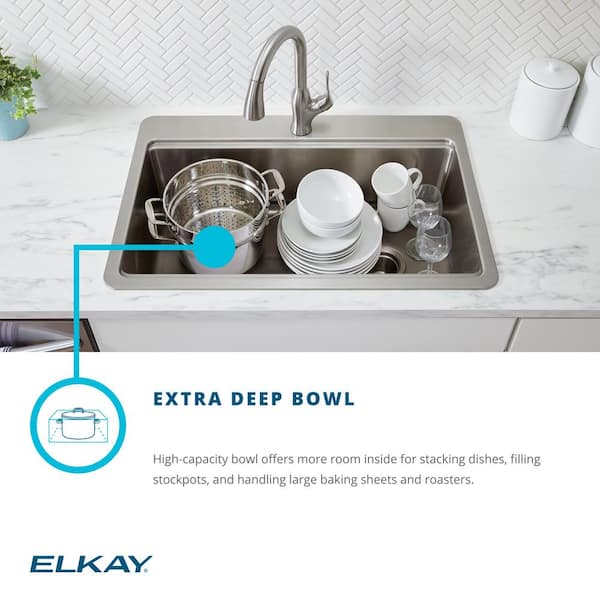The image is a color photograph in landscape orientation, showcasing a kitchen sink advertisement. The focal point is a large, stainless steel, single-bowl sink that is inset into a white marble countertop with gray veins. The sink is filled with stacked white dishes, including plates and bowls, as well as wine glasses, a large silver colander, and a pot. Above the sink, a silver arc faucet adds to the modern aesthetic.

The backsplash behind the sink features a white chevron tile pattern arranged diagonally. To the right of the sink, there are two white canisters, likely for sugar and flour, and to the left, a small green plant adds a touch of color.

At the bottom left of the sink, a blue dot with an arrow points to an enlarged circle depicting a cross-sectional view of the sink, emphasizing its depth. The text in dark blue reads "Extra Deep Bowl," with additional black text stating, "High-capacity bowl offers more room inside for stacking dishes, filling stockpots, and handling large baking sheets and roasters." The brand name "ELKAY" is prominently displayed in italic dark blue letters in the bottom left corner.

Overall, the image highlights the sink's practicality and spacious design, making it ideal for managing large kitchen tasks.